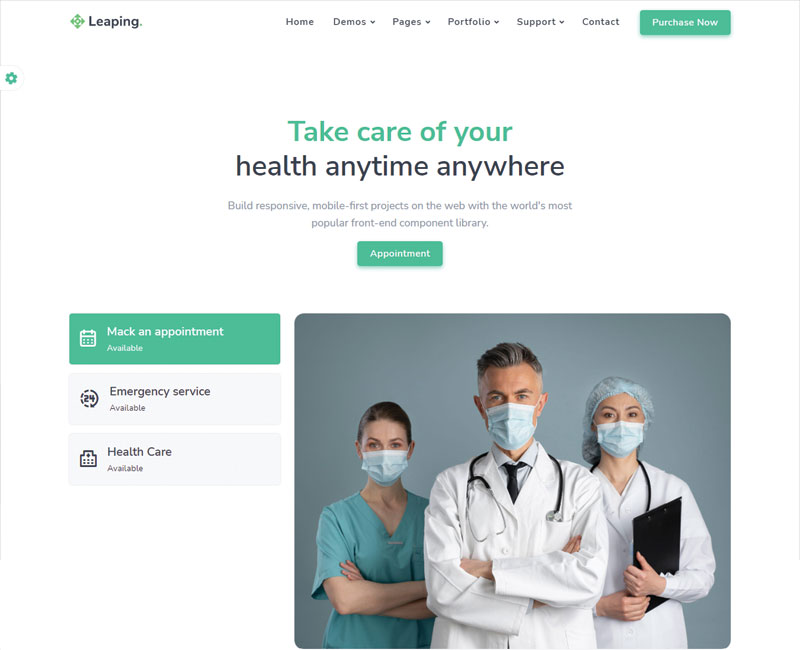The image appears to be an advertisement for a healthcare company, featuring three healthcare workers who are all wearing masks. In the foreground stands a serious-looking doctor with a stethoscope draped around his neck and his arms folded confidently in front of him. Behind him to his right is a woman dressed in white, likely a resident, and to his left, a woman in green who appears to be a nurse or an assistant. The company being advertised is called "Leaping," and it is dedicated to providing healthcare services anytime, anywhere. The website mentioned offers various services including appointment bookings and emergency healthcare. The top navigation bar of the website includes options labeled Home, Demos, Pages, Portfolio, Support, and Contact, with "Purchase New" prominently highlighted in green. Additionally, the website features a settings option for further customization.